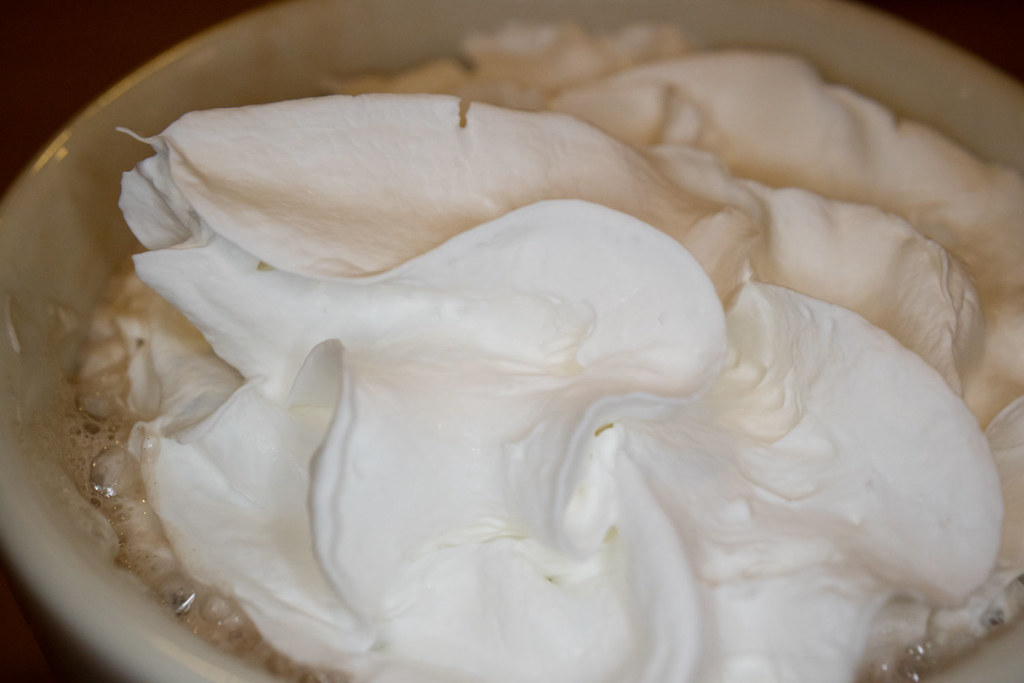The image depicts an extreme close-up of a large, light-colored, circular ceramic bowl, possibly beige or white, containing a food or beverage item. The rear edge of the bowl is out of focus, with a dark background visible in the corners of the image, enhancing the focal point. The contents appear to be a frothy, white mass with folds and curves, suggestive of whipped cream, Cool Whip, or meringue. Parts of the mass are browned, adding texture and depth. Surrounding the edges of the bowl are various-sized bubbles, indicating a liquid or semi-liquid substance beneath the creamy top layer. The overall impression is one of a thick, decadent topping, perhaps on a hot chocolate or a similar warm beverage. The zoomed-in perspective does not reveal the entire bowl, leaving some ambiguity about the exact nature of the vessel and contents.